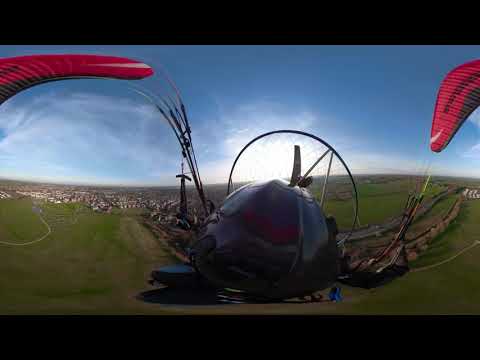The image captures a thrilling viewpoint possibly taken from a helmet camera of an individual engaged in paragliding or parachuting. The wide-angle shot envelops the parachute across the frame, emphasizing its red, wing-like structure extending to the sides. Central to the image is a distinct black helmet, suggesting the presence of the paraglider, who is navigating through the bright blue expanse. The sky features a hazy white area near the center where the sun shines, casting a luminous backdrop. Below, verdant grassy fields and clusters of buildings, hinting at a distant town, are visible, particularly on the left side of the frame. The entire scene is framed with black bars along the top and bottom, enhancing the dramatic perspective. The bright, outdoor setting accentuates the adventurous spirit of the moment, as the paraglider soars high above the landscape, capturing a breathtaking aerial view.